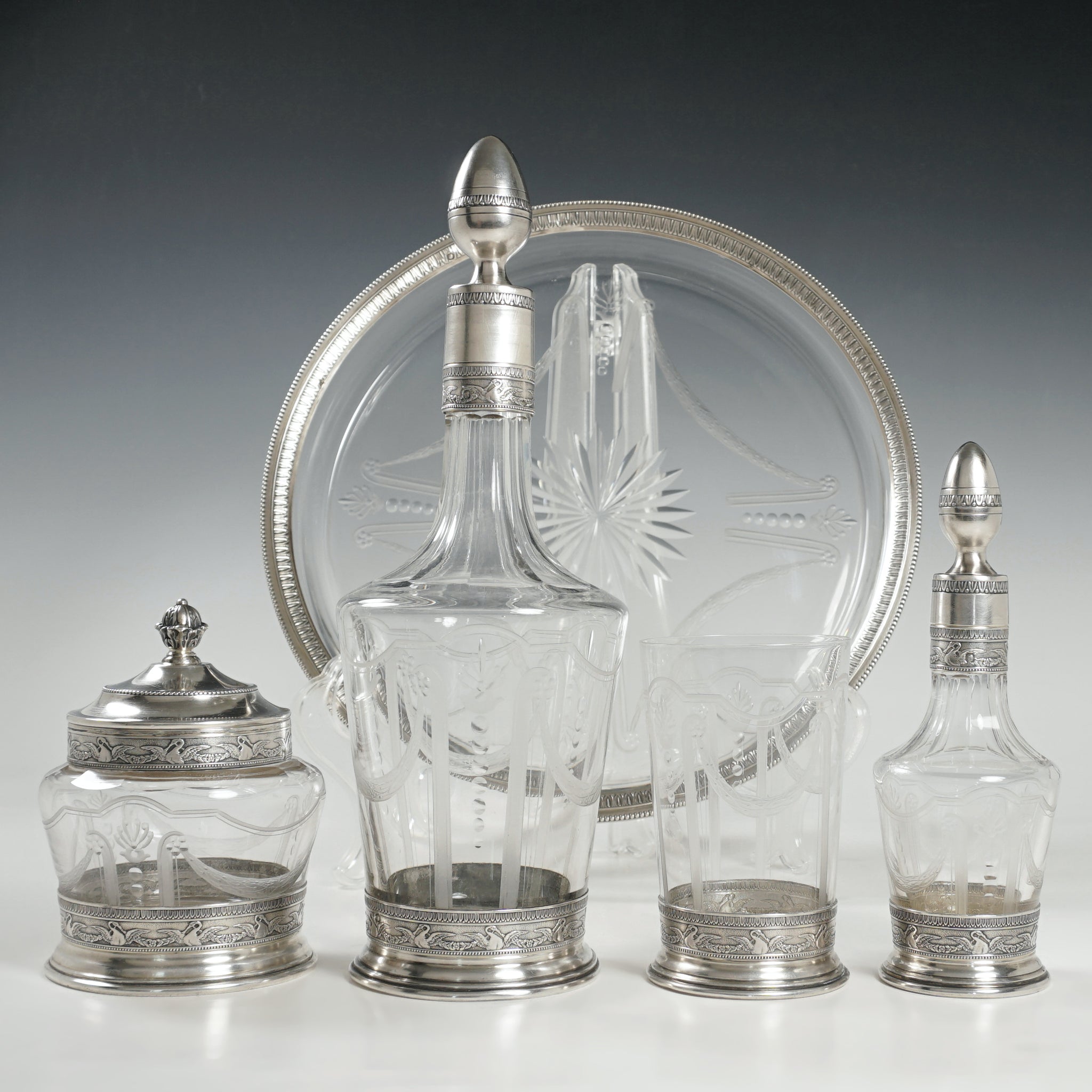The photograph captures an elegant display of antique glassware, meticulously arranged on a white table against a gradient gray backdrop. Central to the scene is a transparent glass plate, held upright, with a silver or metal lining around its border. The plate features a delicate design, possibly depicting two robed figures facing each other in front of a glass starburst. In the foreground, there are four distinct containers, all adorned with ornate sterling silver accents and intricate bird designs etched into their bases. 

From left to right: 
- The first container is short and squat, similar in size to a sugar bowl, with a metal top.
- Next is a tall, thin decanter resembling a wine bottle, characterized by its thick base, slender neck, and an egg-shaped topper.
- Adjacent to that is a small, open glass with a silver-accented base.
- Finally, on the far right, a shorter version of the tall decanter, also featuring an egg-shaped lid, stands gracefully.

The glassware exhibits an exquisite blend of functionality and decorative artistry, evoking a sense of timeless elegance and craftsmanship.